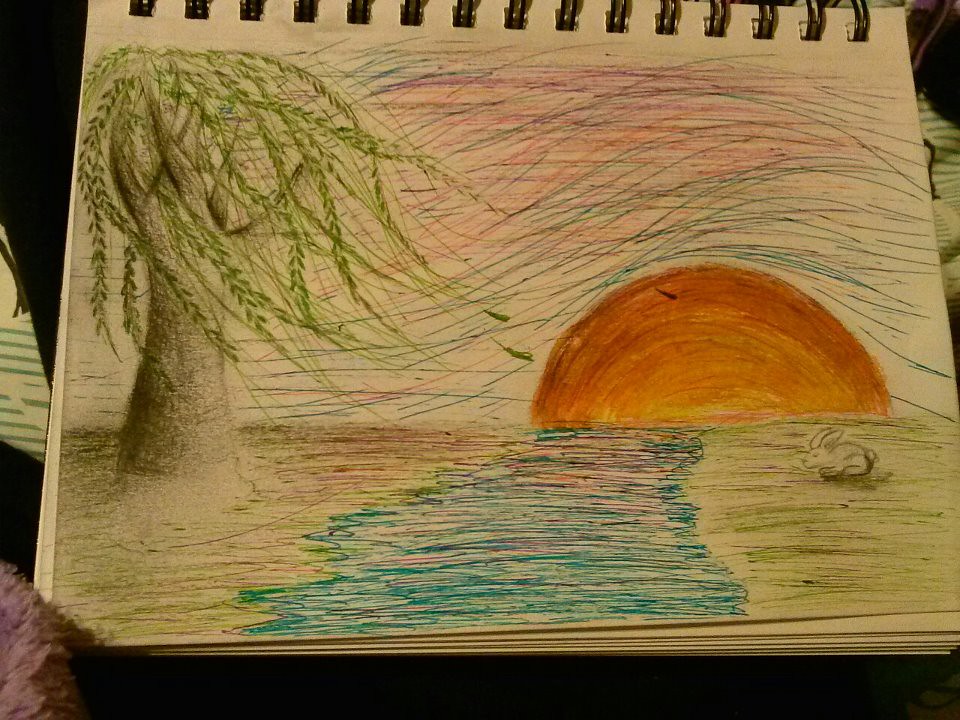A photo taken indoors under regular lighting captures a hand-drawn image on a piece of white or cream-colored paper, housed within a spiral-bound notebook. The artwork features a serene scene with a pastel-hued sky at either sunrise or sunset, displaying a range of soft, rainbow-like colors including magenta, soft orange, and hints of blue. In the foreground, a rabbit stands on a grassy field, separated by a tranquil river or creek from a willowy tree to the left. The bark of the tree showcases intricate shading, indicating the play of light and shadow where the Sun's rays do not directly reach. The rabbit's right side is illuminated by the Sun, while its left side, facing the viewer, is cast in shadow. The entire drawing appears to be meticulously crafted using colored pens or gel pens, adding a vibrant, smooth texture to the scene.